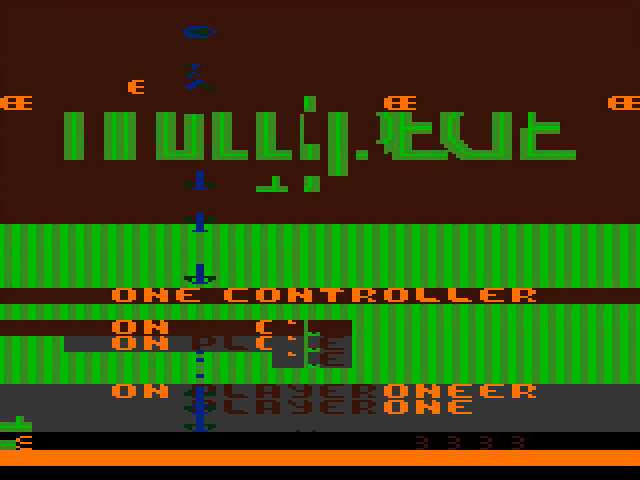The image depicts a pixelated and malfunctioning 8-bit video game screen, likely from an Atari game. The top one-third is predominantly black, with a distorted and incomplete title featuring green letters and blue dashes along the left side suggesting significant video corruption. Amidst the pixelation, faint orange characters are visible, forming sequences like OE, E, OE, and OE. Two horizontal green bands with dark and light green stripes span across the middle of the screen, intersected by a black bar inscribed with "one controller" in orange text. Below this, another black bar carries the word "on," with a subsequent gray line reading "one." Further down, amidst more pixelation, phrases such as "one," "O'near," and "player one" in shades of gray and orange appear, bordered by thin black and orange bars, contributing to the overall disjointed and fragmented look of the image.